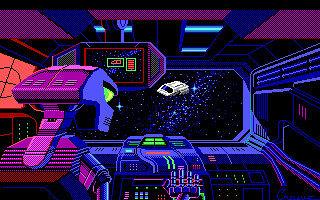The image portrays a scene from a colorful computer game set inside a spaceship. Central to the image is a robot, characterized by a uniquely colored head with a purple front and blue sides. Its eyes are neon yellow and green, adding a vivid contrast. The back of the robot’s neck features a blend of pink and blue shades, while its armor, predominantly purple with red accents and blue outlines, adds to the intricate design.

The robot is intently staring at a complex dashboard, illuminated with a vibrant array of blues, greens, and purples. Beyond the dashboard, the vast expanse of space is dotted with stars, and a spaceship or a similar object appears to be approaching. To the robot’s left, there's a radar screen, glowing in a distinct pinkish-red hue, adding to the high-tech ambiance of the spaceship's interior.